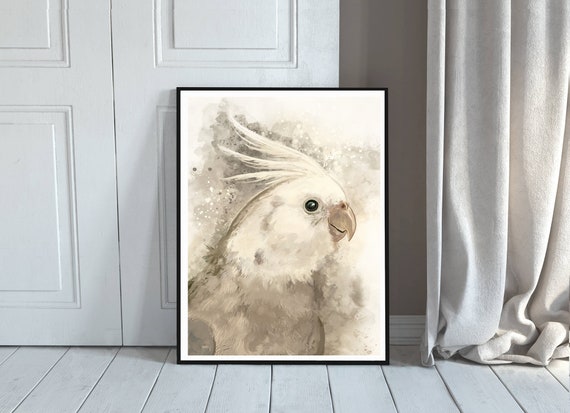The image features a white door on the left-hand side with a design characterized by rectangular panels. Adjacent to the door, the wall is painted a beige tone. The image appears to be zoomed in, revealing a lighter beige material that resembles curtains, though it is not fully clear. On the right side of the door rests a rectangular framed canvas with a black outline and white surface. The artwork depicts a bird with beige, white, and gray plumage. The bird's head is white, turned to the right, showcasing a black eye, beak, and three distinct feathers atop its head.